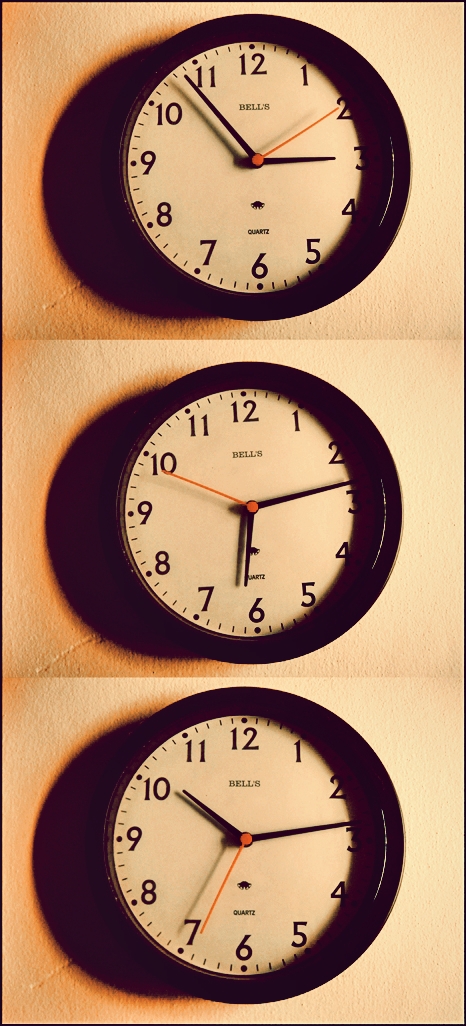This image features three vertically stacked clocks, each divided by a line. Each clock is identical, with a black outer ring, black minute and hour hands, and a red second hand. The clocks are mounted on an off-white wall with a deep crescent-shaped shadow to the left, reminiscent of a moon's shadow with an opening towards the right. The clocks display the name "Bells" at the top and "Quartz" at the bottom center, with standard block numbers in regular order. The times displayed are 2:54 on the top clock, 6:13 on the middle clock, and 10:14 on the bottom clock.